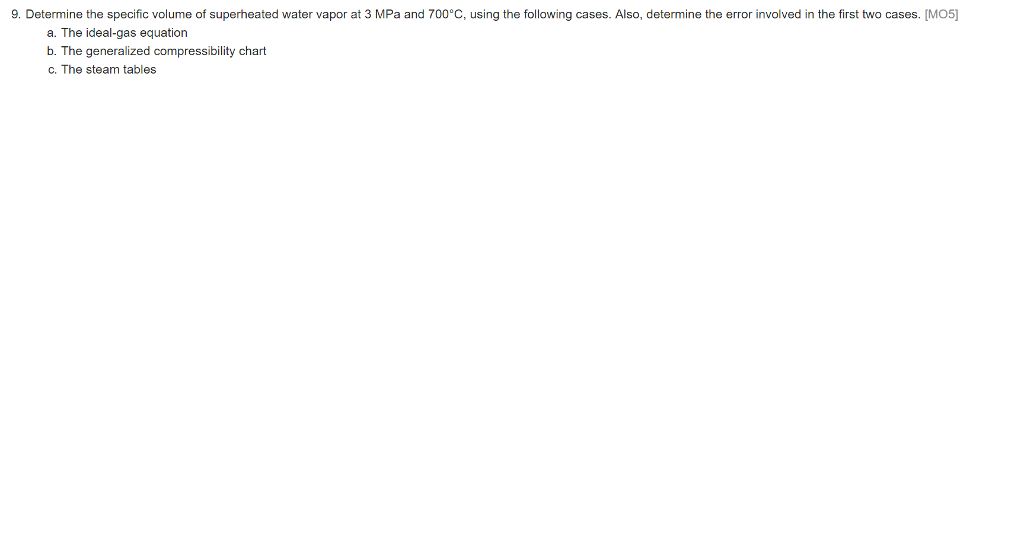**Caption:**

The image features a minimalistic design with a plain white background. At the top, the number "9." is prominently displayed in dark lettering, which appears to be either black or dark blue. Adjacent to this, the following directive is written:

"Determine the specific volume of superheated water vapor at 3 MPa and 700°C using the following cases. Also determine the error involved in the first two cases. [M05]"

Beneath this instruction, the image enumerates three specific methods, each marked by a lowercase letter in dark blue lettering:

a. The ideal-gas equation.

b. The generalized compressibility chart.

c. The steam tables.

These instructional elements are clearly organized and color-coded for readability and emphasis.